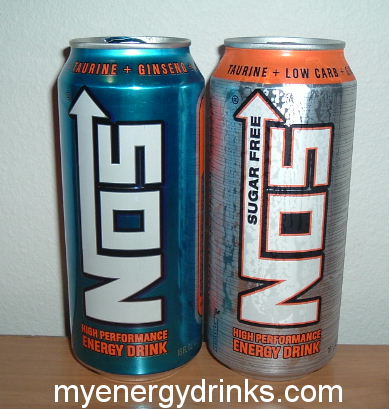The photograph showcases two prominent cans of energy drinks positioned on a brown surface against a stark white wall. Each can is emblazoned with the brand name "N05" and the phrase "High Performance Energy Drink" at the bottom. The can on the left is primarily blue, highlighted with orange text reading "Taurine + Ginseng" and the name of the drink in bold white letters. Adjacent to it, the can on the right is predominantly silver, marked with "Sugar-Free" on the brand name. This silver can features an orange section at the top and contains the text "Taurine + Low Carb," although part of the text on this can is obscured and unreadable.